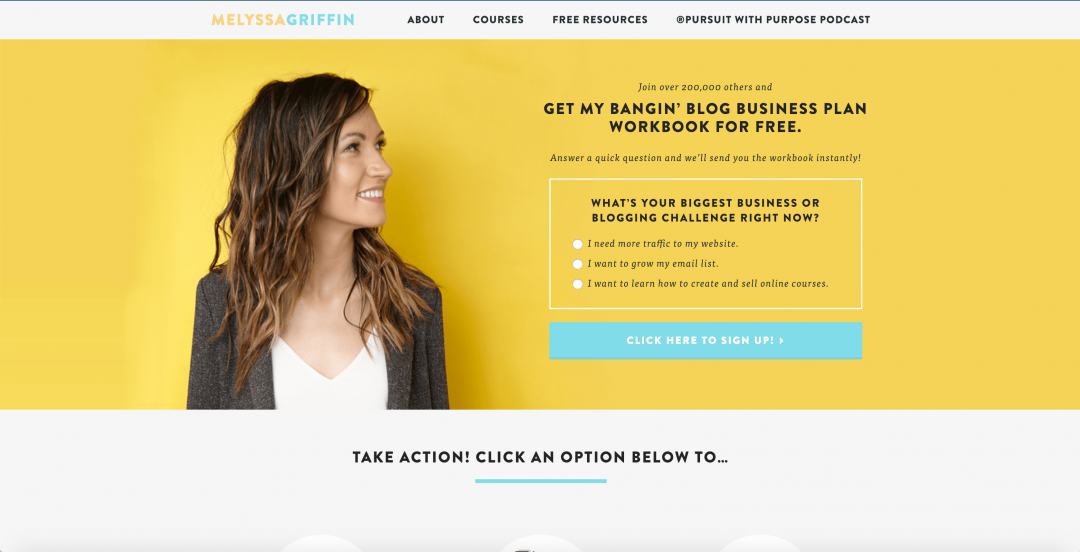This is an image of Melissa Griffin's website. The top menu bar, with a gray horizontal background, features navigation items including Courses, Free Resources, and the Pursuit with Purpose podcast. To the left of the menu bar, "Melissa" is uniquely spelled as "Melyssa" in a vibrant yellow font, while "Griffin" is displayed in an aqua font.

Directly beneath the menu bar, there is a bold yellow background stretching across the width of the page. On the left side of this background, there is an image of a woman. She stands facing forward, but her head is turned to the right, capturing just the profile view of her face. She has brown hair and is dressed in a gray blazer or sweater over a white top. She smiles gently as she looks towards a section on the right side of the yellow background.

In this section to the right, there is a promotional text stating, "Get My Blogging Business Plan Workbook for Free." Below this text, there is a prominently placed button inviting visitors to "Click Here to Sign Up." The overall design is clean and inviting, effectively drawing attention to the available resources and the action call for signing up.